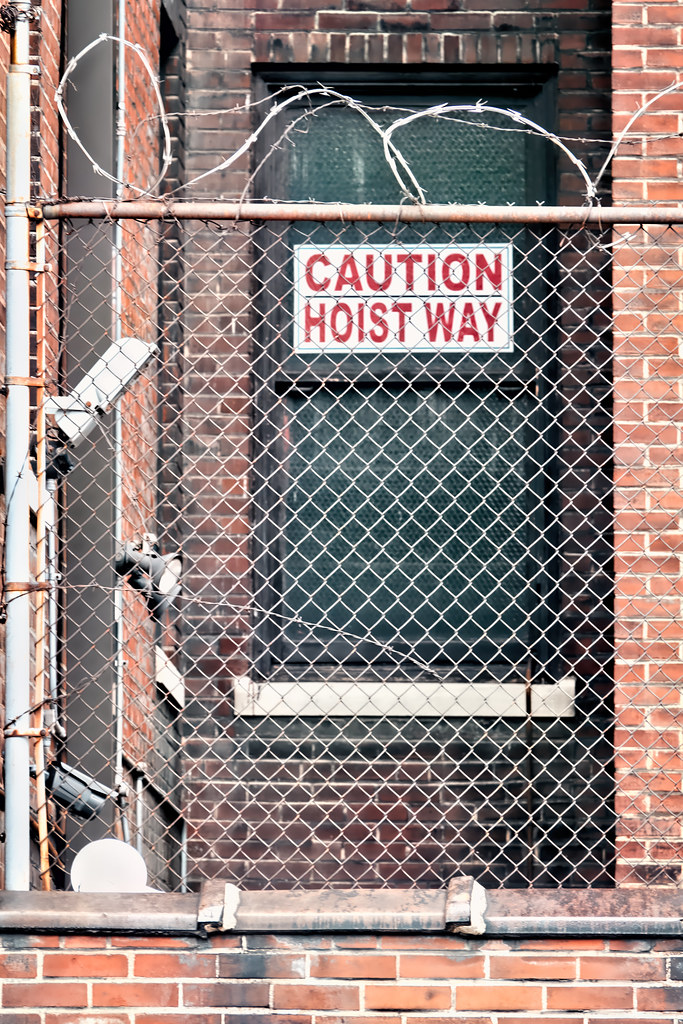This full-color photograph captures a scene in daylight, depicting an aged brick building in what appears to be a city location. Dominating the foreground is a chain-link fence topped with razor wire, positioned in front of a window. The window displays a white sign with red lettering that reads "Caution: Hoist Way." Around the base and surroundings of the structure, the bricks show considerable wear, appearing singed and very old, potentially hinting at a history involving heat or fire. To the left of the fence, a metal rod is visible, and scattered bits of metal adorn the area, contributing to the gritty, industrial atmosphere. Additionally, some fixtures, which could be lights or cameras, are observable on the structure. The overall composition highlights the interplay of deteriorated materials and protective barriers, evocative of a setting steeped in industrial purpose and urban character.